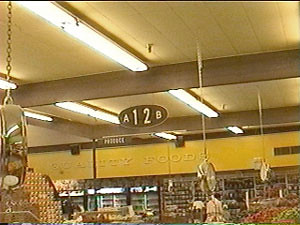The image depicts a nostalgic, possibly vintage-styled photograph of the interior of a grocery store, emphasizing the ceiling with its intersecting brown beams and fluorescent lighting tubes. The ceiling and walls exhibit an array of yellow and brown hues, reminiscent of a retro 1970s aesthetic. Hanging from the ceiling, a sign reads "A12B," with a barely discernible "produce" sign beneath. The background features a golden-colored wall adorned with the words "Country Foods" or "Quality Foods" in a retro font. Below are cases and coolers, along with indistinct images of food items and some stacked cans. A shiny silver scale can be seen hanging from the ceiling, and a few figures of shoppers are visible amidst the produce, primarily red and green, further contributing to the busy atmosphere of the grocery store.